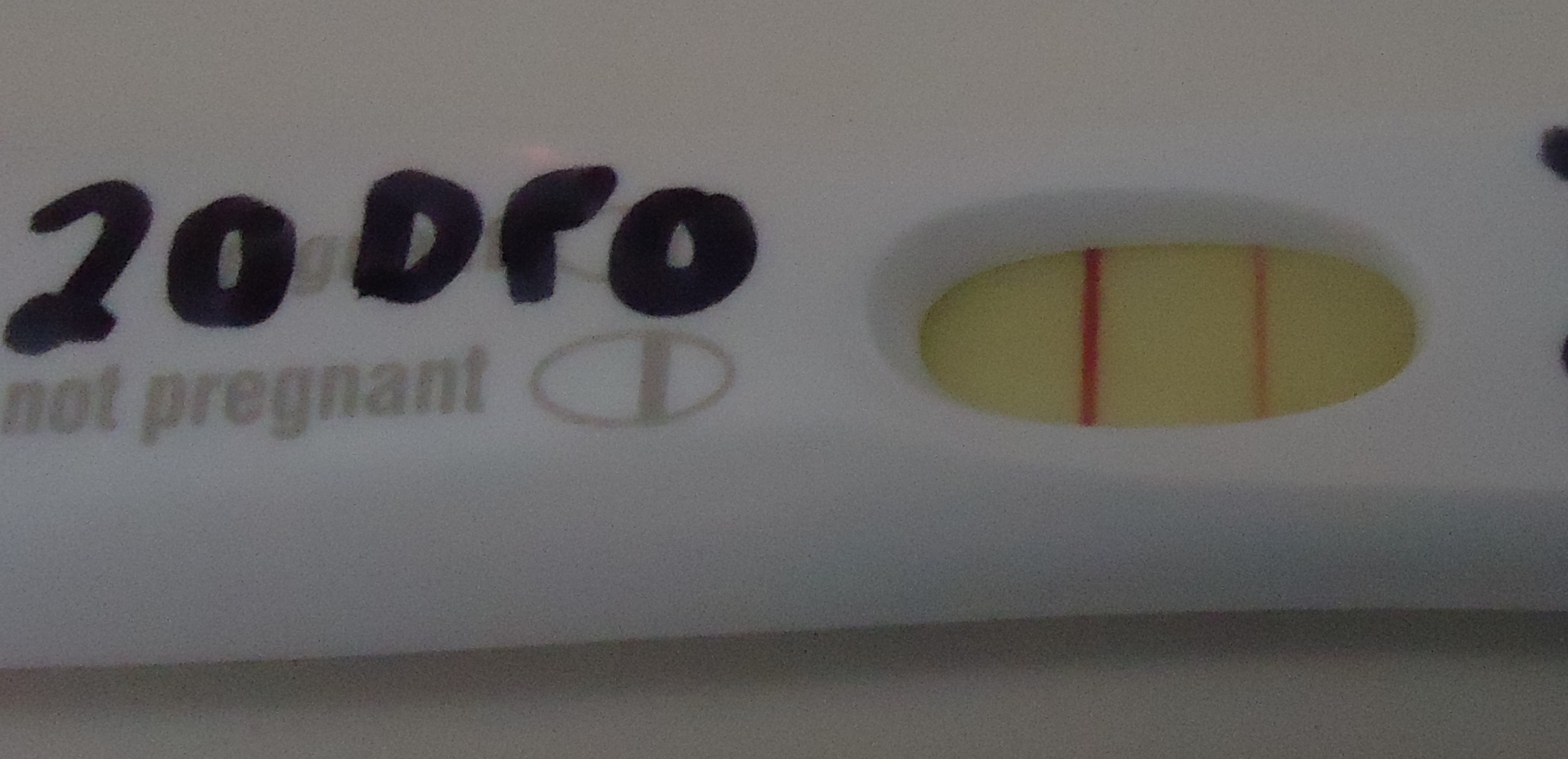This close-up image captures a pregnancy test resting on a white table, filling the entire frame. The test itself is a white plastic device with an oblong window displaying the results. Inside this window, there appears to be yellow-tinted litmus paper showing one bright red line and a second, fainter red line. Above the window, the words "Not Pregnant" are printed in gray on the plastic, along with a reference image indicating what the result lines would look like, showing one thick line. The top of the test also features handwritten text in black marker, reading "20 DPO." A subtle shadow is cast beneath the test onto the table. Additionally, there are hints of more black marker writing to the right of the test window, though only part of the lettering is visible and illegible.